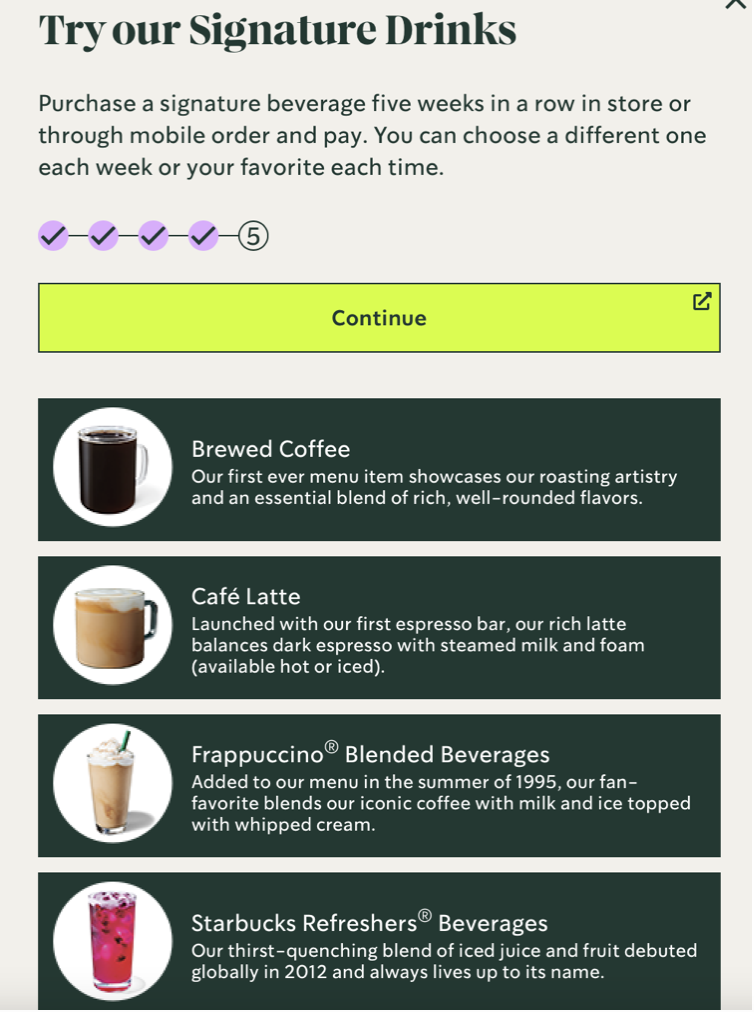The promotional image features an aesthetically pleasing background and prominently displays a call-to-action saying, "Try our signature drinks" in bold black text. The highlight of the image is a promotional offer: purchase a signature beverage in-store or through mobile order and pay for five consecutive weeks to qualify. Participants can choose a different drink each week or stick with their favorite. The progress is tracked with five circular icons; the first four circles are purple and checked off in blue, while the fifth circle is blank with a number "5".

Below the promotional offer, there is a detailed description of four signature beverages presented in blue rectangular sections:

1. **Brewed Coffee**: Described as the first-ever menu item, it highlights their roasting artistry with a blend of rich and well-rounded flavors.
2. **Cafe Latte**: Launched as part of their finest espresso bar, this beverage features a perfect balance of dark espresso, steamed milk, and foam. It is available both hot and iced.
3. **Frappuccino Blended Beverages**: Introduced in the summer of 1995, this fan-favorite blends coffee with milk and ice, topped with whipped cream.

At the bottom of the image, a green rectangle marked "Continue" directs viewers to proceed further. In the top right corner, a square with an arrow points diagonally upwards to the right, hinting at progress or advancement.